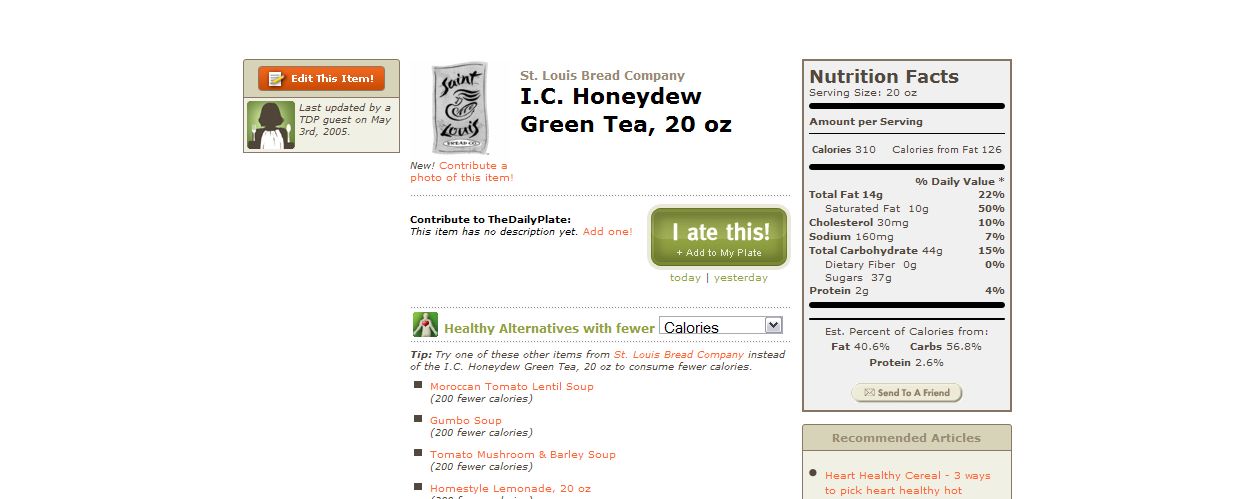This detailed caption describes an image displaying nutritional information for a product named "I.C. Honeydew Green Tea," produced by St. Louis Bread Company. The image seems to be from a review or nutrition tracking site, possibly viewed on a computer. The left side of the image features the St. Louis Bread Company logo, alongside text indicating "edit this item" with a notepad icon, and the note "Last updated by TDP guest on May 3rd, 2005."

Prominently to the right, there is a rectangular box containing the full nutritional facts for the 20-ounce beverage, featuring details such as 310 calories, 14 grams of total fat (including 10 grams of saturated fat), 30 milligrams of cholesterol, 160 milligrams of sodium, 44 grams of total carbohydrates (37 grams of which are sugars), and 2 grams of protein. Below the nutritional facts, the text "recommended articles" is noted.

Additionally, a green rectangle in the image states "I ate this," with options to "Add to my plate" for "Today, yesterday." It also mentions "Healthy alternatives with fewer calories," suggesting trying other St. Louis Bread Company products like soups or lemonade instead of the "I.C. Honeydew Green Tea" to consume fewer calories.